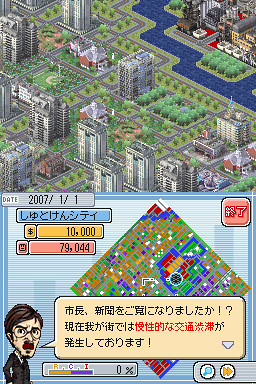The image consists of two distinct panels, seemingly from a video game. The top panel showcases a detailed rendering of a small city. Dominated by gray buildings interspersed with green grass and roadways, the cityscape features strategically placed green bushes. A narrow waterway, resembling a river or canal, divides the land, creating an island that occupies the upper right corner of the panel. This island boasts a dense arrangement of yellow, brown, and white structures, hinting at a bustling community.

The bottom panel appears to be a game board, likely representing the city from a tabletop game perspective. This overhead view is vibrantly color-coded with red, blue, green, white, yellow, and orange squares that layout the city’s plan. Various informational boxes, which are color-coded in yellow, blue, and pink, are adorned with text in an unknown language. A peach-colored text box suggests speech or dialogue. In the lower left corner of this panel, stands a small human character with distinct features: brown mustache and short brown hair, light skin, dark-rimmed glasses, and a dark long-sleeved shirt.